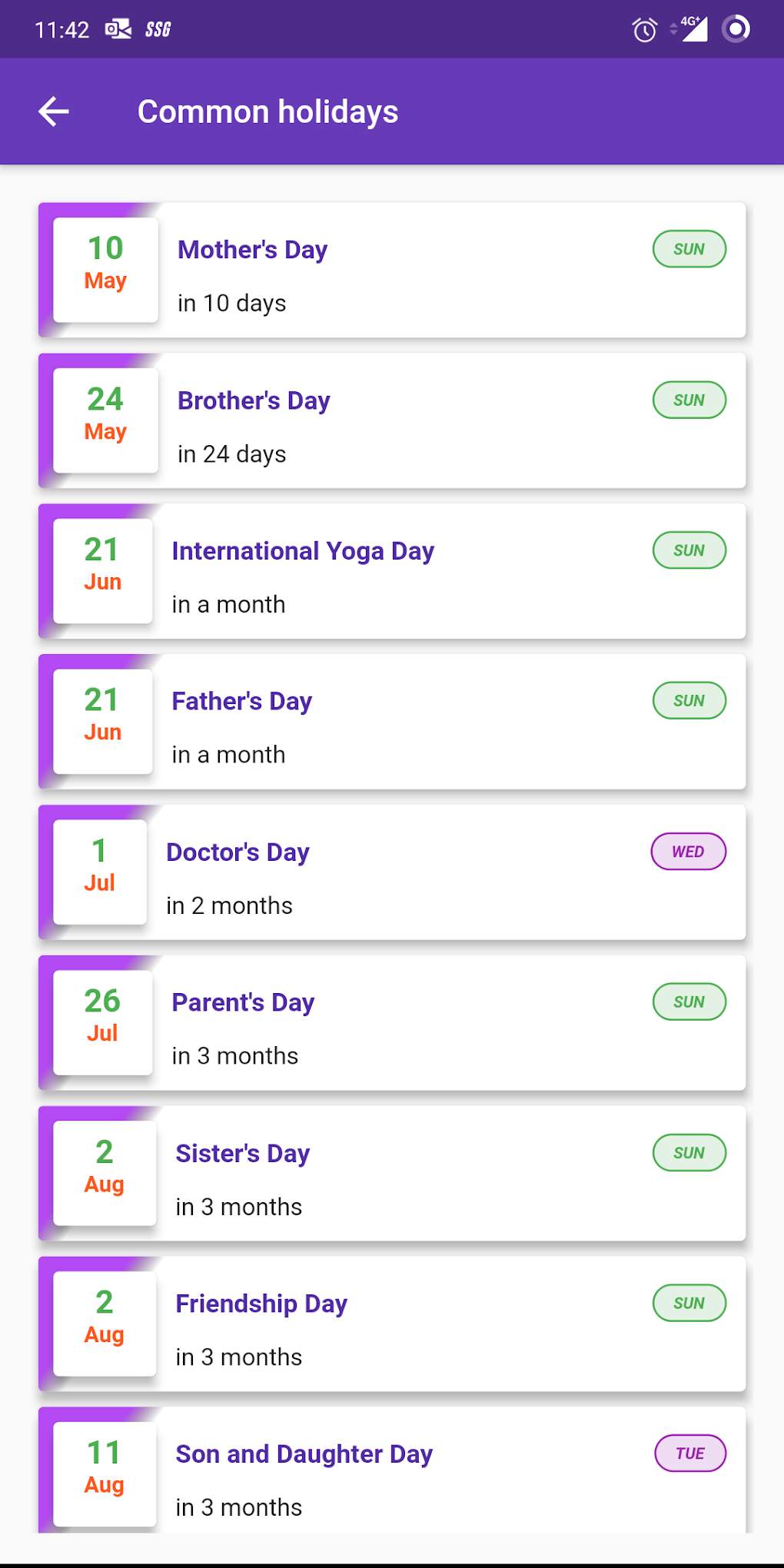The image is a screenshot of a website or app displaying a list of upcoming holidays. At the top, it prominently features a section titled "Common Holidays." Below this heading, the holidays are listed with their respective dates and a countdown to each:

- **Mother's Day**: May 10th, in 10 days
- **Mother's Day**: May 24th, in 24 days
- **International Yoga Day**: June 21st, in about a month
- **Father's Day**: June 21st, in about a month
- **Doctor's Day**: July 1st, in two months
- **Parents Day**: July 26th, in three months
- **Sister's Day**: August 2nd, in three months
- **Friendship Day**: August 2nd, in three months
- **Son and Daughter Day**: August 11th, in three months

On the right side of the image, there are small bubbles indicating the day of the week each holiday falls on. All the holidays are on a Sunday except for:

- **Doctor's Day**: Highlighted in purple, lands on a Wednesday
- **Son and Daughter Day**: Highlighted in purple, lands on a Tuesday